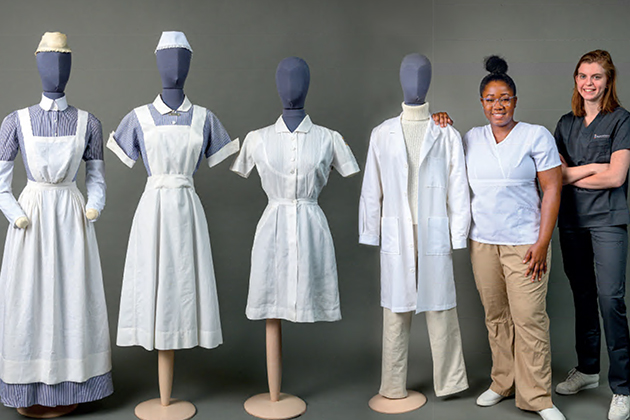The image presents an evolution of nurse uniforms over time, featuring a variety of styles displayed on both mannequins and live models against a gray background. On the far left, a gray mannequin is adorned with a blue and white striped long-sleeve dress extending to the ankles, paired with a white apron and a white hat. Next to it, another mannequin showcases a similar ensemble but with short sleeves and a knee-length dress, accentuated by a wider cap. The third mannequin displays a white dress with front buttons that is cinched at the waist. The fourth mannequin wears a turtleneck sweater under a white medical coat, complemented by tan pants. On the right side of the image, two live models stand, each showing a modern variation of nurse uniforms. The first model, with reddish hair, sports a gray uniform with white shoes. The second model, a black woman with her hair in a bun, wears a white short-sleeve shirt and tan pants. The distinct contrast between the historical and modern uniforms, as well as the diversity in their presentation, highlights the transformation in nursing attire over the years.